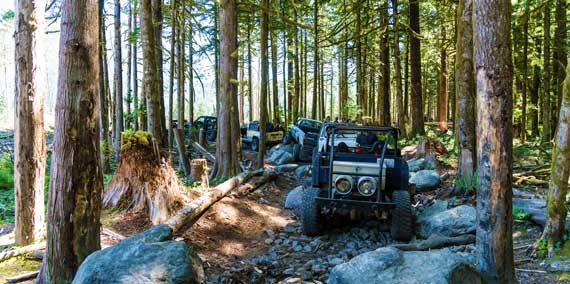The photograph captures a vibrant daytime scene set in a dense forest with tall trees featuring brown trunks and green leaves. The forest floor is rugged, characterized by a rocky dirt pathway that meanders through the trees. Along this stone-laden trail, multiple off-road vehicles, including open-roof Jeeps or trucks, are lined up, navigating the uneven terrain. Some vehicles have visible drivers. On the left side of the trail, a few tree trunks have been cut down, leaving only stumps behind, with the surrounding soil appearing brown. White daylight filters through the canopy, enhancing the bright and clear ambiance of the outdoor environment.